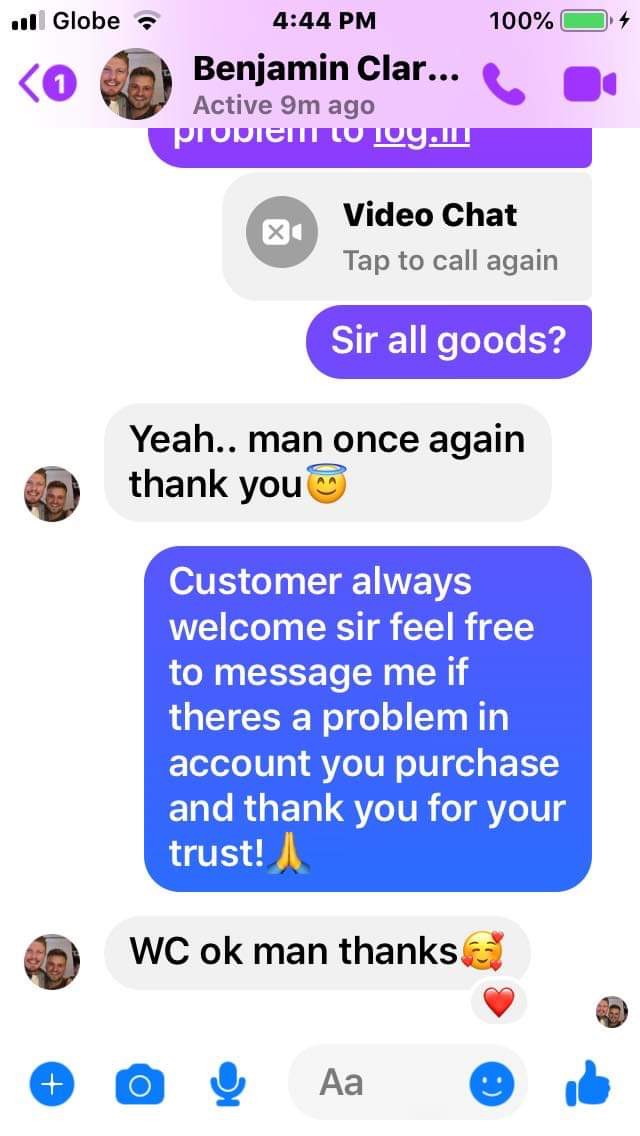The image is a screenshot capturing a text conversation between two individuals using a messaging application that resembles WhatsApp. At the very top of the screen, the status bar includes signal bars with a globe icon at the center, the time "4:44 PM," and a green battery icon indicating 100% charge. To the right, the contact name "Benjamin Clare" appears, followed by an "Active 9m ago" status, and icons for phone and video calls, as well as a back arrow. 

Just below, a circular avatar shows two smiling white men, with the taller one on the left. The initial message from the seller, appearing on a bluish-purple background, reads, "Sir, all good?" The customer responds on a white background with, "Yeah, man. Once again, thank you," accompanied by a smiley face emoji with a halo.

Following this, the seller's message on a blue background says, "Customer always welcome, sir. Feel free to message me if there's any problem with the account you purchased. Thank you for your trust," and includes a praying hands emoji. The customer replies on another white background with, "OK, man, thanks," adding an emoji with a smiling face surrounded by hearts and a heart emoji below.

At the bottom of the screen, various chat buttons are displayed, including icons for a camera, a plus symbol, a microphone, a smiley face, and a thumbs-up, all in blue against a predominantly white background.